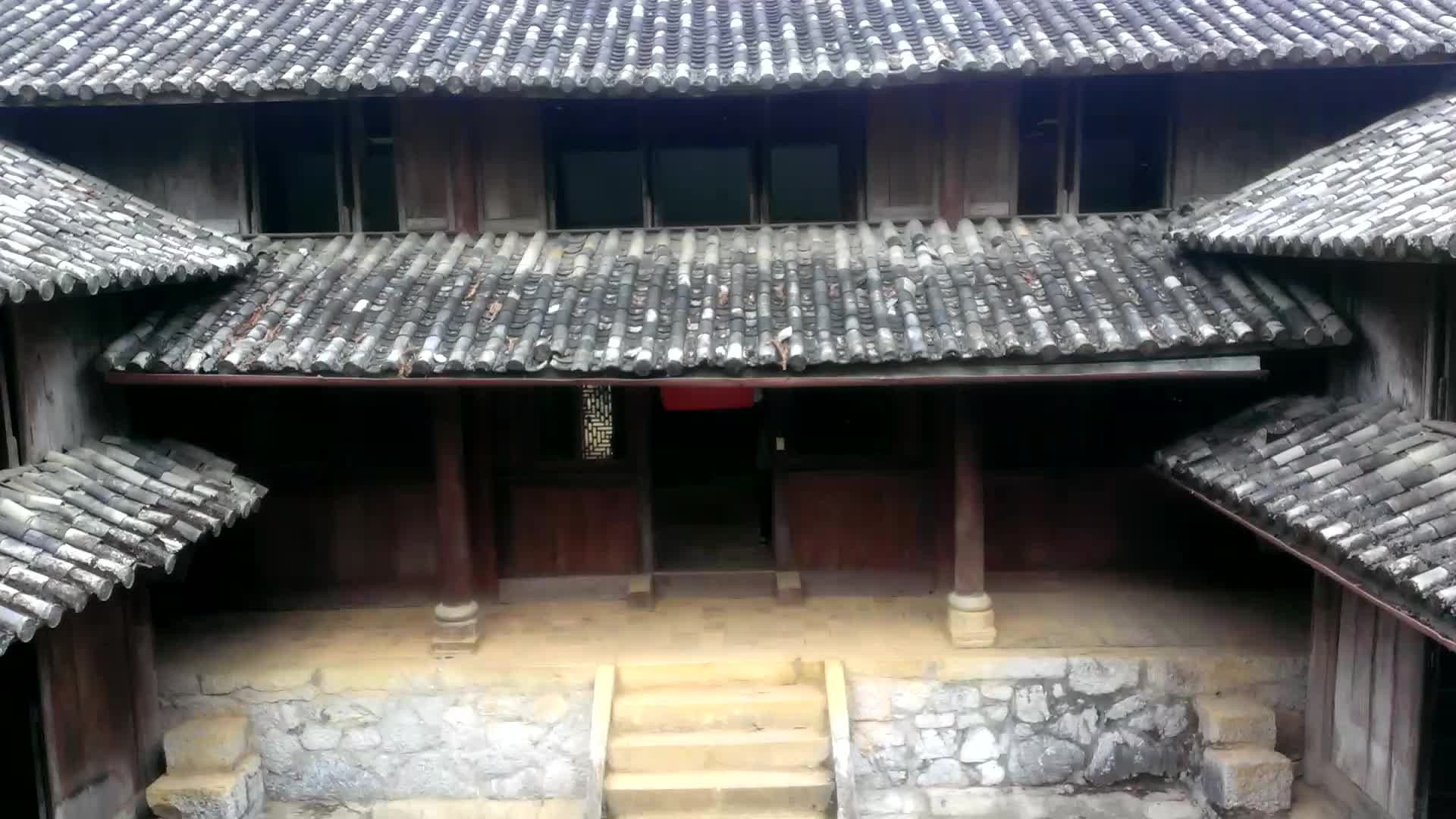This image captures a detailed view of an Asian, possibly Chinese temple or building, framed by a courtyard. The structure occupies the entire screen, showcasing its traditional architectural elements. The main entrance is centered with a small door, flanked by two wooden posts. A set of light-colored stone steps leads up to a stone porch, which is similarly light in color. The porch features an awning supported by the posts, offering a welcoming shade. 

The building is two stories tall, with the first story painted a darker brown and the second story a lighter gray, nearly white. Adjacent to the main building are two symmetrical two-story wings, noticeably shorter in height due to their lower rooflines. The roofs, made of black tiles with some white accents, resemble long narrow tubes placed next to each other, a characteristic feature of traditional Asian roofing. 

The upper story of the central structure houses three windows; the middle one is larger than the two flanking it. Similar roof awnings are present on both stories, lending a layered appearance to the architecture. The area around the steps is bordered by small rock walls, enhancing the rustic, harmonious feel of the temple grounds.